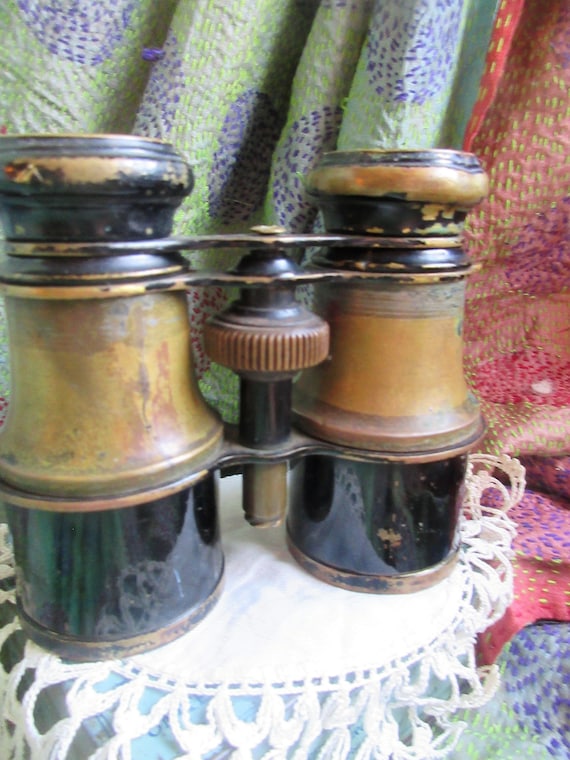A vivid photograph captures a vintage pair of metal binoculars, predominantly black with scuffed gold accents and some rust, indicating their age and frequent use. The binoculars, shorter and compact in design, rest atop a small table adorned with a delicate white doily-like tablecloth featuring intricate patterns. This table is part of a cozy, well-lit room where the white tablecloth contrasts strikingly with the surrounding colorful textiles. Behind the binoculars, the backdrop is a charming assortment of colorful fabrics and quilts, including a green and blue patterned quilt and one with pink, yellow, and lavender circles. A green curtain with blue designs and a red-colored or multicolored curtain further enhance the room’s vibrant ambiance, making the binoculars the focal point of this artistic and potentially commercial image.